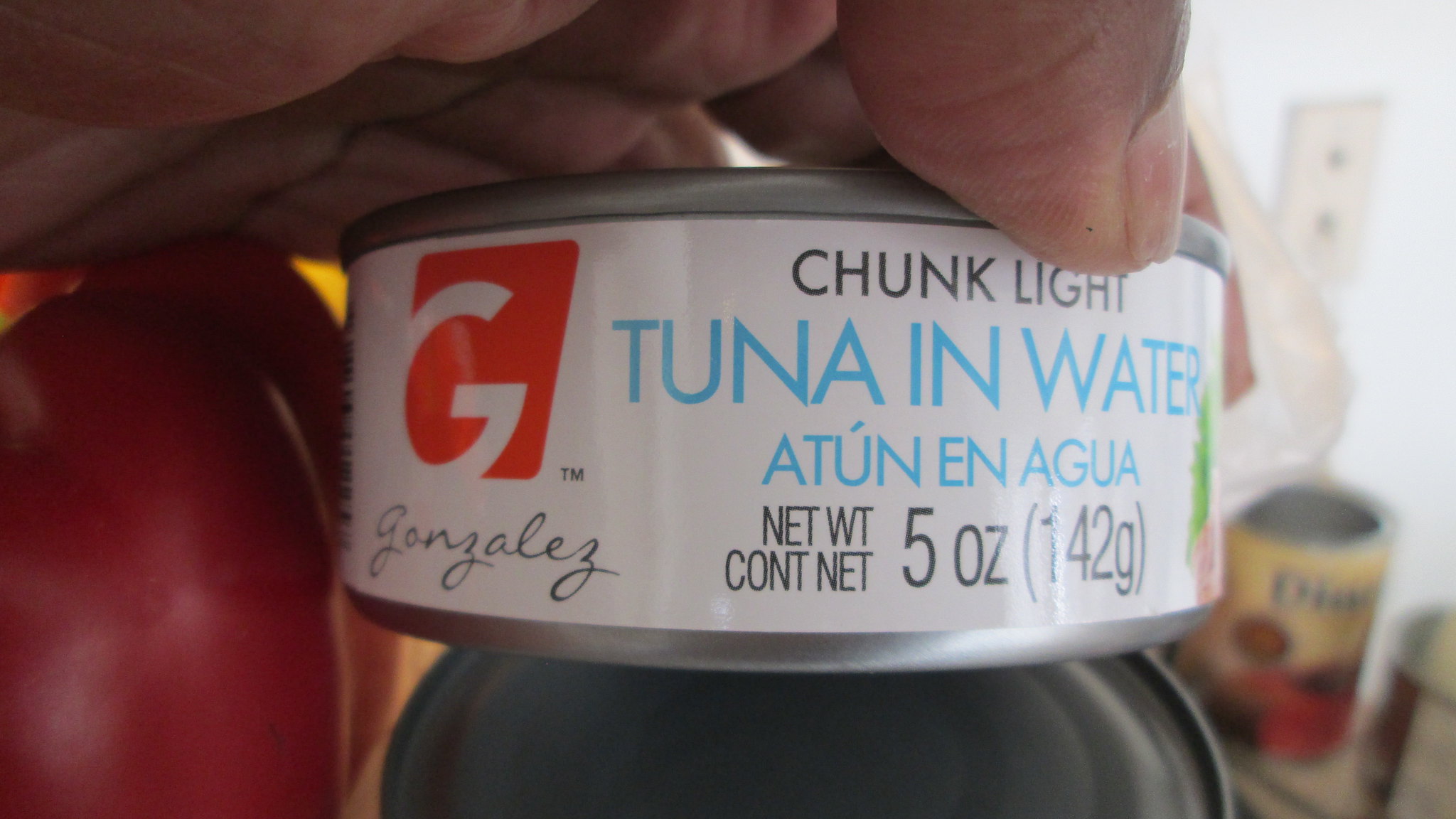The close-up photograph depicts a person's hand holding an aluminum can of tuna, displaying intricate details of its labeling. The can, adorned with a white paper label, prominently features a red "G" logo and the brand name "GONZALES." Written in black text, the label reads "CHUNK LIGHT," followed by "NET WEIGHT 5 ounces (142 grams)." In light blue text, it indicates "TUNA IN WATER," which is also repeated in Spanish as "Atún en Agua." The can, visibly small and round, is being held in place by the individual's fingers, partially obscured from view. Beneath the can, another tuna can is perceptible, and to the left, a hint of a red pepper (mistaken for a red paper in one description) is visible, adding a pop of color to the image. The setting appears to be kitchen-like, with a secondary mention of other items such as cans of tomatoes or an apple to the left, suggesting a casual and everyday environment.